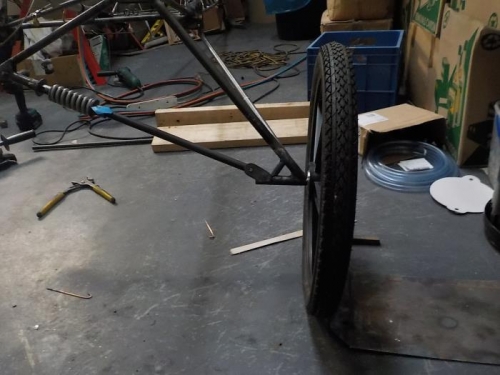In the image, a mechanical contraption is prominently displayed on what appears to be a grease-laden, dirt-smudged surface that could either be an old, weathered tabletop or a floor. Central to the contraption is a bicycle tire, which is affixed via a pivot featuring a spring, suggesting a flexible joint. This arrangement implies the tire might be part of a larger mechanism, possibly a wagon or another wheeled vehicle. Surrounding the contraption, there are various tools and materials indicative of a tinkerer’s workshop environment. 

Directly behind the vehicle is a set of wire cutters, and further back, a wooden frame becomes visible. Coiled plastic tubing and a blue box containing white material, potentially made of plastic or metal, are also scattered around the work area. The background reveals more of the vehicle’s frame, made of black metal with two connection points—one rigid and the other designed for flexibility, possibly featuring a coil or pneumatic element. The setting, with its array of equipment and the evident signs of wear and tear, paints a vivid picture of an active DIY enthusiast's workspace, immersed in ongoing projects and mechanical explorations.